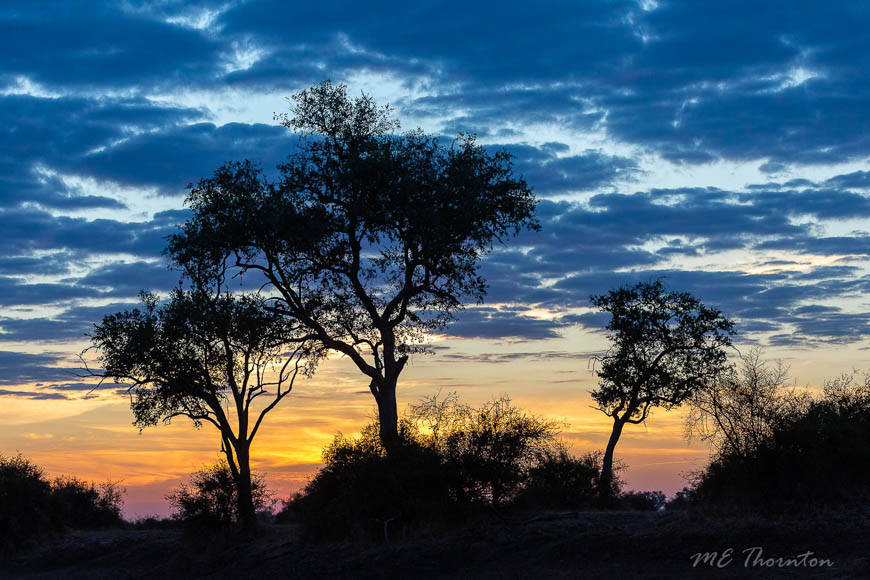This stunning photograph captures the serene beauty of a sunset sky, with the lower right-hand corner bearing the signature "M.E. Thornton" in white lettering, denoting the photographer. The scene features a natural landscape comprised of a mix of trees, bushes, and patches of grass. Three prominent trees stand out against the horizon: one on the left, one on the right, and a taller one in the middle, their branches gracefully framing the sky. The sunset imbues the clouds with a breathtaking palette of orange, yellow, pink, and purple hues. These colorful clouds contrast vividly with the clear blue sky above, dotted with white clouds, creating a mesmerizing and tranquil vista.